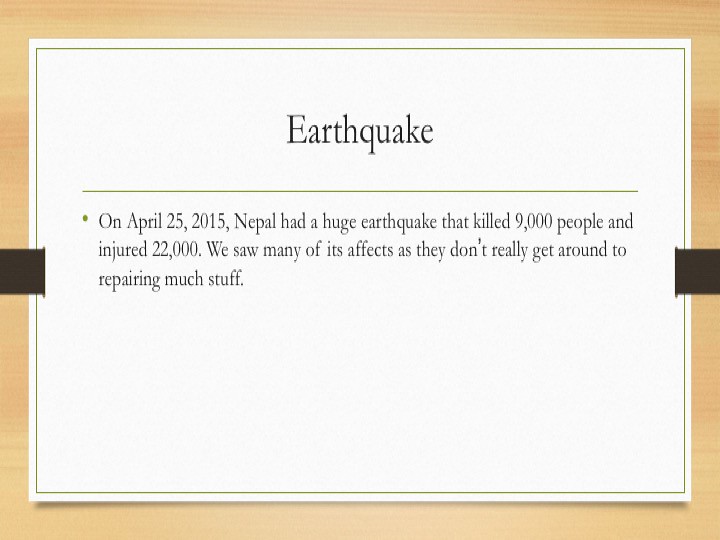The image features a digital depiction of a white piece of paper that appears to be taped to a wooden board. The entire composition is framed by an orange border. Along the left and right sides, centered, are decorative black squares. Centered on the white paper, the word "earthquake" is prominently displayed in bold black letters, with a thin green line underneath it. Below this, a green bullet point precedes the text: "On April 25th, 2015, Nepal had a huge earthquake that killed 9,000 people and injured 22,000. We saw many of its effects, as they don't really get around to repairing much stuff." This summary provides an impactful reminder of the earthquake's devastating aftermath.